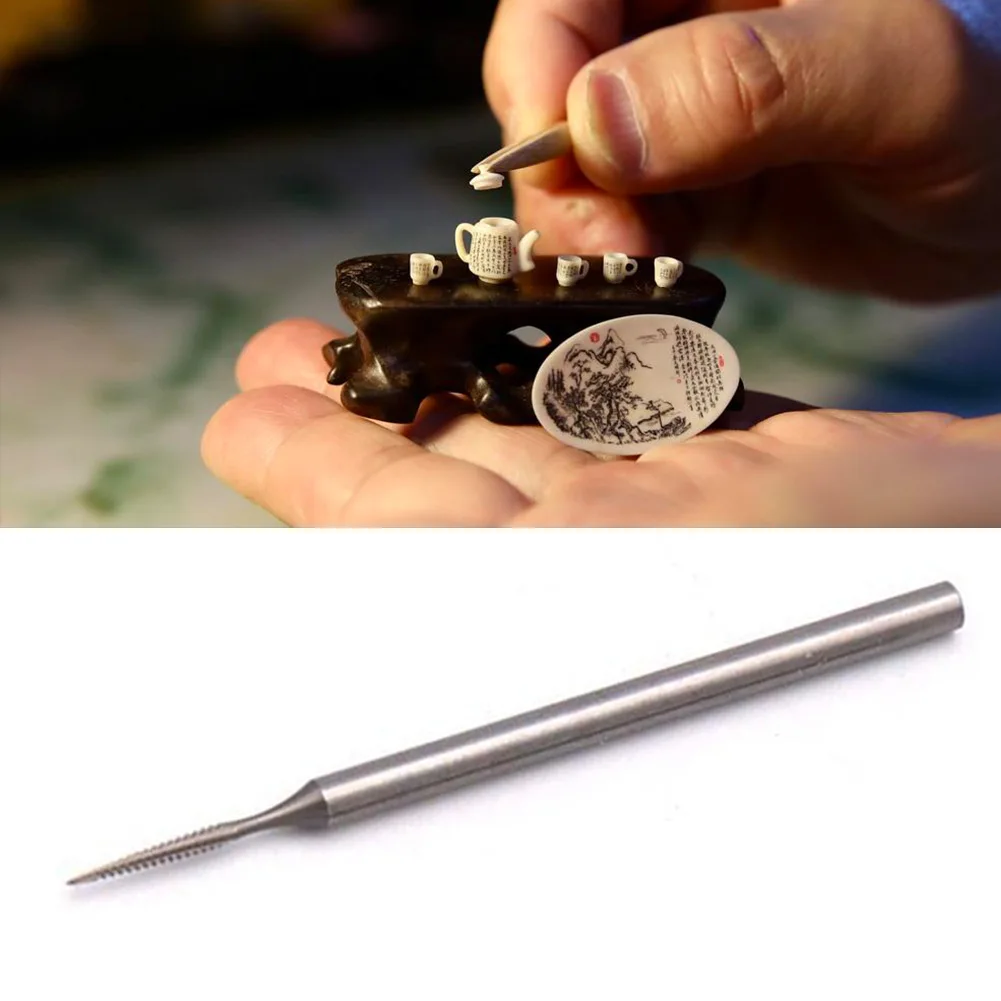The image features a split composition with a top and bottom section, with each part rich in detail. The top half centers on a miniature wooden table set with a meticulously carved tea set, including a tea kettle and several small cups, all adorned with Japanese symbols. The objects are so small that a person's hand, using tweezers, delicately holds the tiny lid of the tea kettle above the table. Another hand rests below, providing a staged platform that supports the miniature setup. 

In front of the table, there's a small, oval-shaped plate decorated with images of mountains and trees, also featuring Japanese lettering. This entire intricate scene is set in colors of grey, peach, blue, white, black, and red, contributing to its detailed aesthetic. 

The lower part of the image features a diagonally placed shank milling cutter, a silver, pen-like woodworking tool with a sharp edge used to craft the miniature tea set. This detailed craftsmanship and the use of varied tools highlight the precision and intricate artistry involved in creating such small objects.